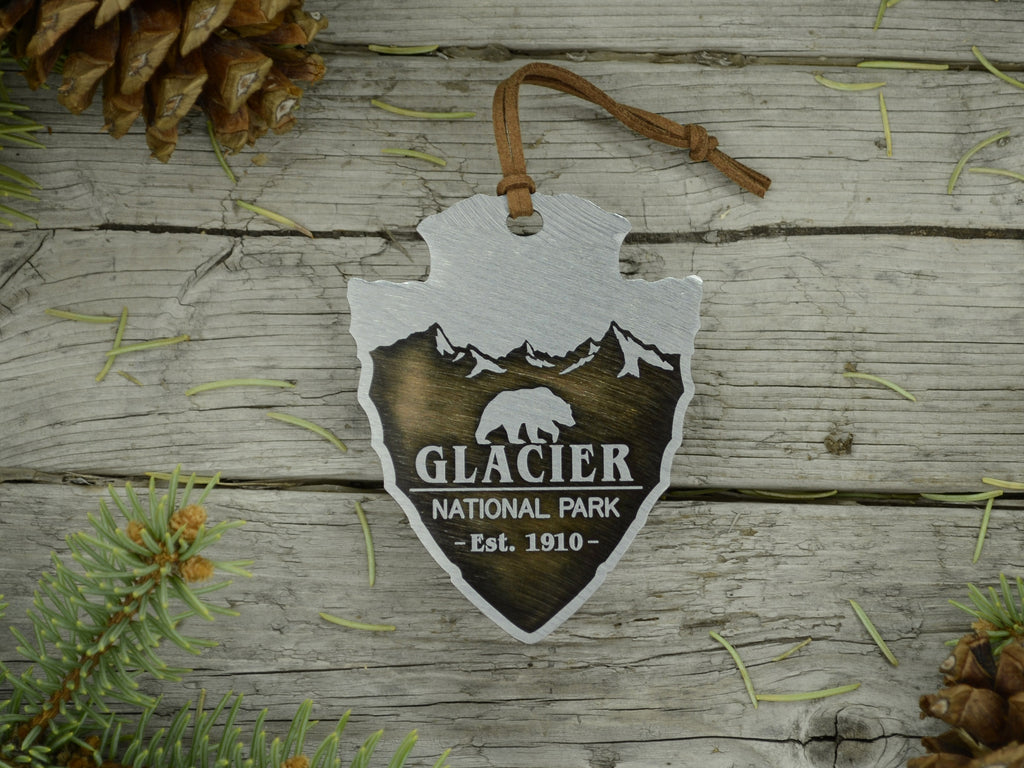The photo is a close-up, outdoor image of a keychain or charm shaped like an arrowhead, showcasing the text "Glacier National Park, established 1910." The charm features a graphic depiction of black mountains with a bear profile walking from left to right above the word "Glacier." The medallion is crafted from a material that appears either metallic or stone-like, with a light gray and dark brown color scheme. It has a hole at the top, through which a leather thong with a knotted tassel is looped. The charm is centrally placed on an aged, light gray-brown wooden bench with visible cracks. The setting includes natural elements such as pine cones and evergreen needles, with a pine cone situated in both the top left and bottom right corners, while the evergreen branches and scattered needles complement the rustic wooden surface.